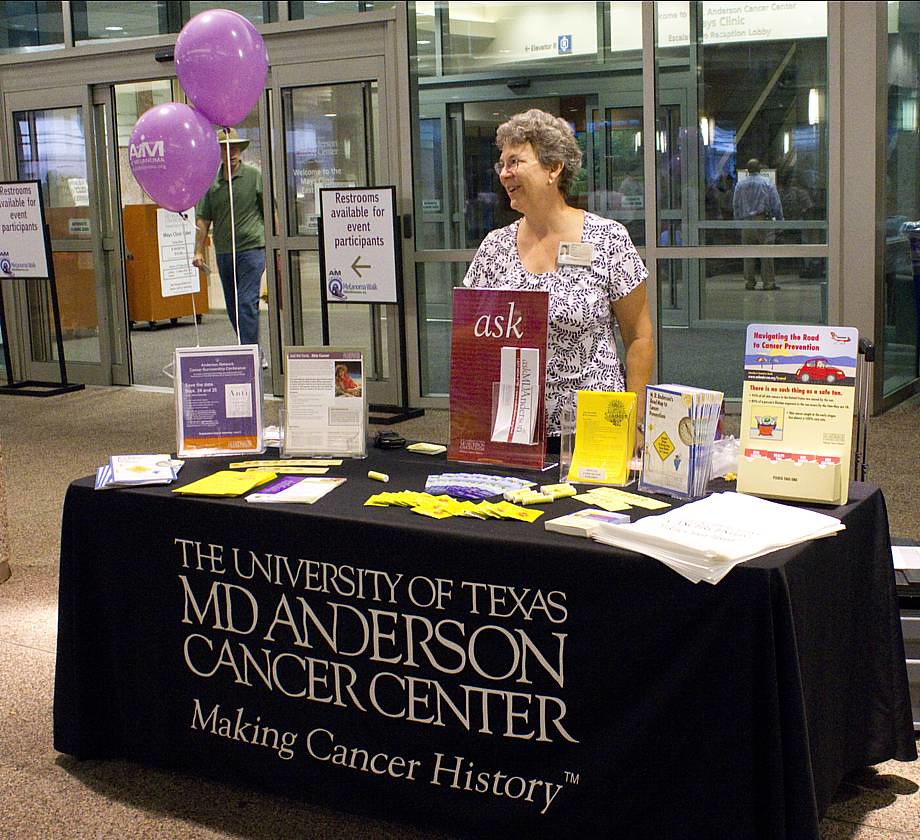In this large, square photograph, an older woman with short, curly brown and white hair stands smiling behind a black tablecloth-covered table. She wears glasses and a name tag on her black and white short-sleeve shirt. The tablecloth prominently displays the text: "University of Texas MD Anderson Cancer Center, making cancer history." The table in front of her is cluttered with a multitude of brochures, some encased in plastic, yellow cards or ticket stubs, small giveaway items, and a stack of papers on the front right corner. To the left of the table, two purple balloons with white writing float cheerfully. The scene is set on a pebbled walkway defined by brown and black speckles. The background features an entrance to a building with large, glass sliding doors and brown-bordered windows. Signs in front of the doors guide event participants to restrooms. The woman looks off to the left, possibly engaged with passersby.